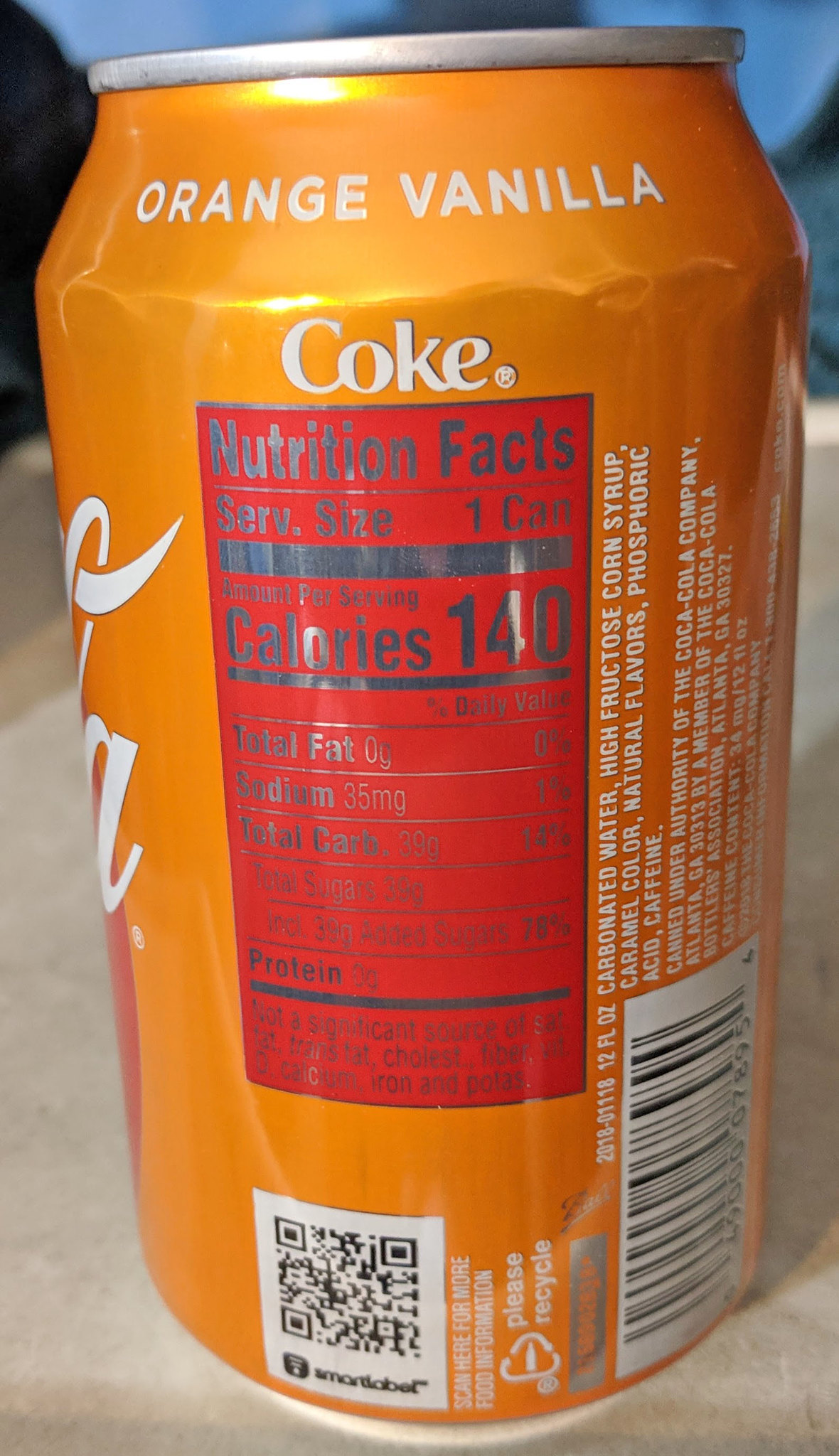This image features a profile view of an orange Vanilla Coke can, prominently displaying its nutrition fact panel. The can, which has a striking light orange hue and a silver top, is labeled "orange vanilla coke" in white letters at the top. The nutrition fact panel on the side is red with gray letters and numbers detailing the usual nutritional information such as serving size, calories, and fat content. At the bottom left of the panel, there is a distinct white QR code with black markings, adjacent to which is a sideways white text that reads "please recycle." To the right of the QR code, as the can curves away, appears a black-barred UPC code on a white background and additional ingredients listed in white. The partially visible Coca-Cola logo in white curvy letters can be seen on the left side of the image. The background comprises a blend of white and black elements, with a hint of blue and a white tablecloth providing contrast.